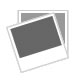The image features an old, rusted metal object lying on a blue, slightly wrinkled tablecloth. At the bottom of the image, a measuring tape is visible, indicating the object is about 10 inches long, with measurements starting at 1 inch on the right and extending to 11 inches. The main metal object has a straight, thinner section on the left, which gradually becomes thicker towards the right. On the right end, there's a bolt where something appears to be attached. Above this attachment point, a curved hook extends upward with a small bend at its tip.

This object closely resembles a fro, a tool historically used in logging. Typically, a fro comprises an iron or wooden shaft inserted into an iron head. The head usually features a missing spike, with a barbed hook designed to dig into logs, enabling loggers to control or roll the logs, especially in water. Despite the wear and rust, the object retains the characteristic hook and broader end, indicative of its use in forestry. Although now obsolete, the fro's design remains a testament to its functionality and application in historical logging practices.